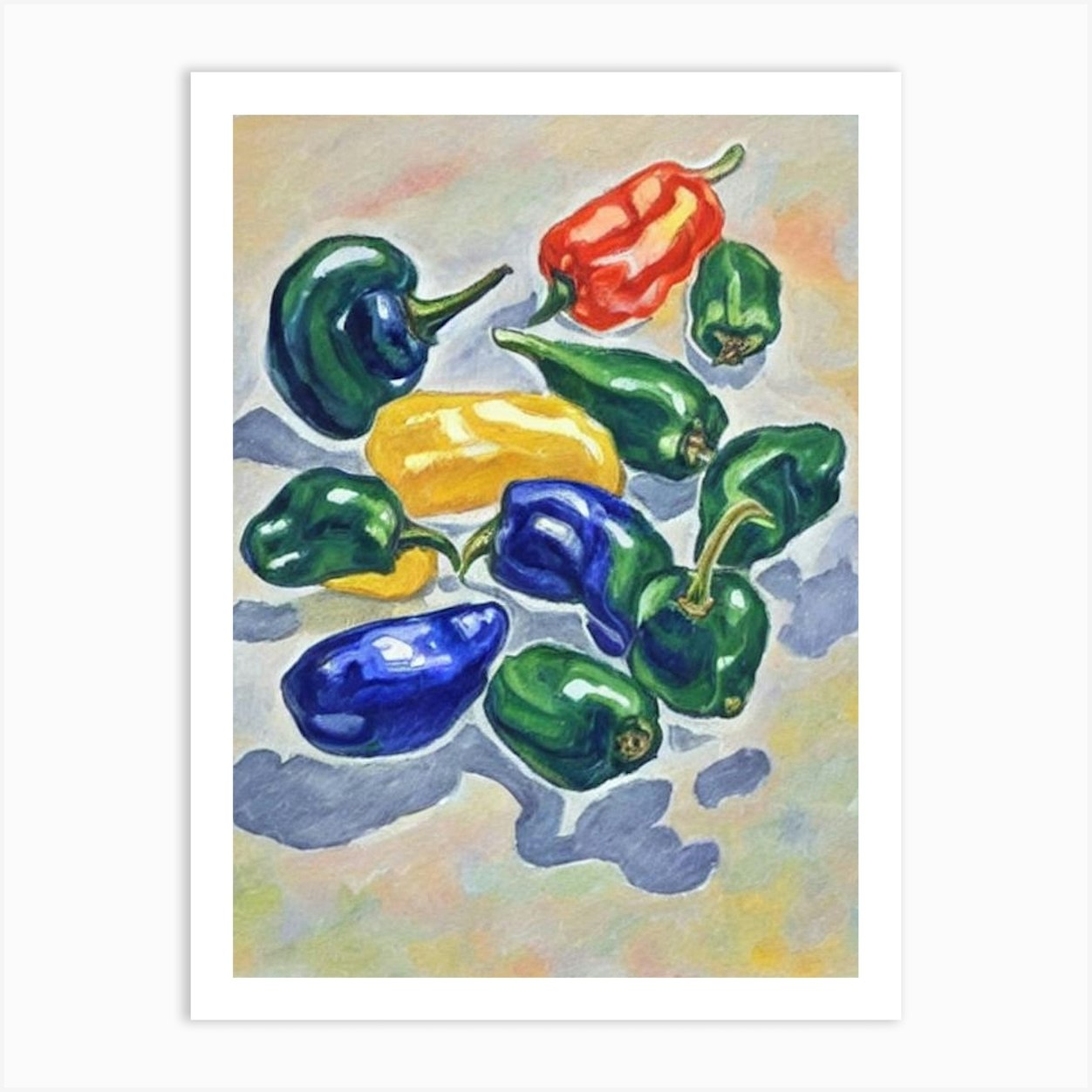This image depicts a detailed watercolor painting set against a white background with a white border surrounding the artwork. The painting showcases a lively assortment of peppers in varied hues and arrangements. At the heart of the composition, a vivid yellow pepper stands prominently, encircled by several green, lumpy-shaped peppers. Also present are two striking blue peppers, an uncommon sight, adding a unique touch to the array. Above the central yellow pepper, there is a red pepper. The background features muted gray tones blended seamlessly with hints of tan and very light orange, providing a subtle contrast that highlights the vibrant colors of the peppers. The overall arrangement of the vegetables appears spontaneous, almost as if they've naturally settled into place, each one casting a soft shadow beneath it. The composition is simple yet engaging, with no text or signature visible, leaving the focus solely on the art itself. It's an interesting piece that intriguingly captures the beauty of everyday produce through the fluid medium of watercolor.